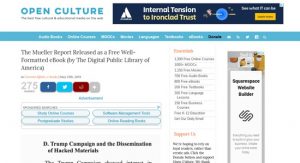This is a detailed screenshot of the OpenCulture website's homepage. At the top left corner, the website's name, "OPENCULTURE," is prominently displayed in blue, all capital letters. Directly beneath the name is a small thumbnail image, further supplemented with text in small black letters that are illegible due to their size. Adjacent to the website's name, is a navy blue rectangular box featuring a white pyramid-shaped logo on its left side. Next to the logo, the phrase "Internal Tension to Ironclad Trust" is written. Continuing to the right, there is a blue circle followed by additional text that is also unreadable due to its small size and a tiny yellow clickable box at the top.

Below this section is a teal-colored horizontal rectangle offering various clickable options, all labeled in white text that is too small to decipher. Further down, there is a section with bold black text, again too small to be read, followed by multiple smaller options underneath it. The dense layout and small font sizes make it challenging to read the detailed content. This detailed description encapsulates the structure and visual elements present on the OpenCulture homepage as displayed in the screenshot.